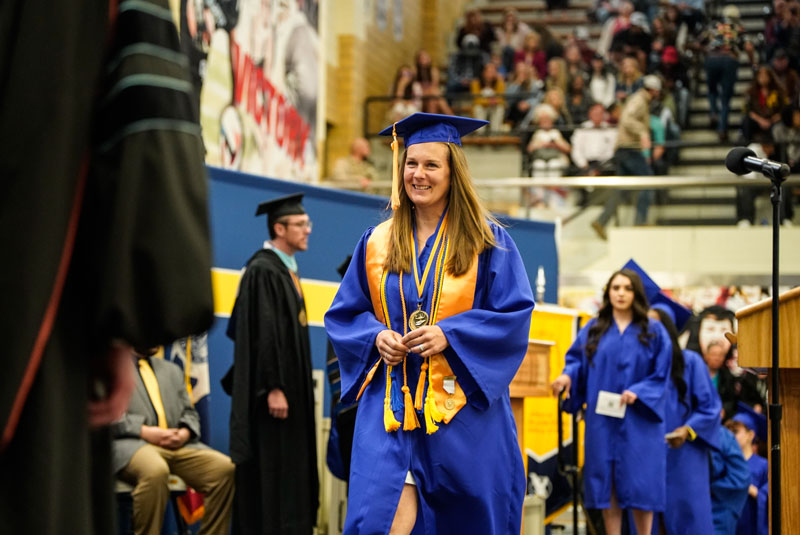This photorealistic graduation image captures the moment from behind a professor or administrator in a black robe with red lettering, positioned in the left-hand corner. At the center, a smiling middle-aged white woman with shoulder-length brown hair stands out in her bright blue graduation gown and cap adorned with a gold tassel. She wears a yellow and blue medal ribbon around her neck, a yellow scarf-style tassel, and other tassels draped over her gown. Her hands are almost interlapsed as she approaches the stage to receive her diploma.

Around her, there's a row of graduates lined up, eagerly waiting their turn, including another brunette woman directly behind her. On stage to the left, additional administrators in black robes await to greet the graduates. The background, slightly out of focus, reveals an attentive audience in the upper right, and the blue wall of the auditorium features some yellow decorations and painted images. A microphone is also visible on the right-hand side, ready for the next announcement.